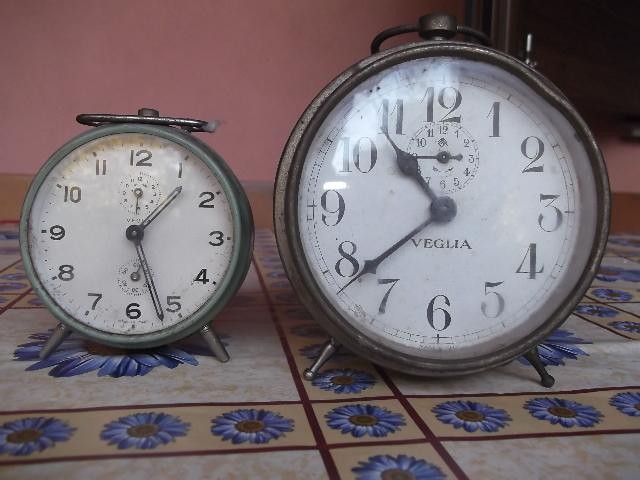This is a detailed photograph showcasing two vintage metal alarm clocks, each with a distinctive character. Both clocks have circular faces with black numbers and hands set against white backgrounds, accented by silver objects on top and sturdy silver legs for support. Resting on a tiled surface with a brown and tan stripe pattern adorned with blue floral motifs, these clocks exude an antique charm. The larger clock, with an aged silvery hue, is slightly dented on its right side and displays the time 10:38. The smaller clock has a greenish tint to its border and is set to 1:27, featuring two additional smaller gauges, likely for seconds. A brand name, "VEGLIA," is delicately inscribed on one of the clock faces. Both clock faces are encased in glass, reflecting a subtle white sheen, hinting at the passage of time.